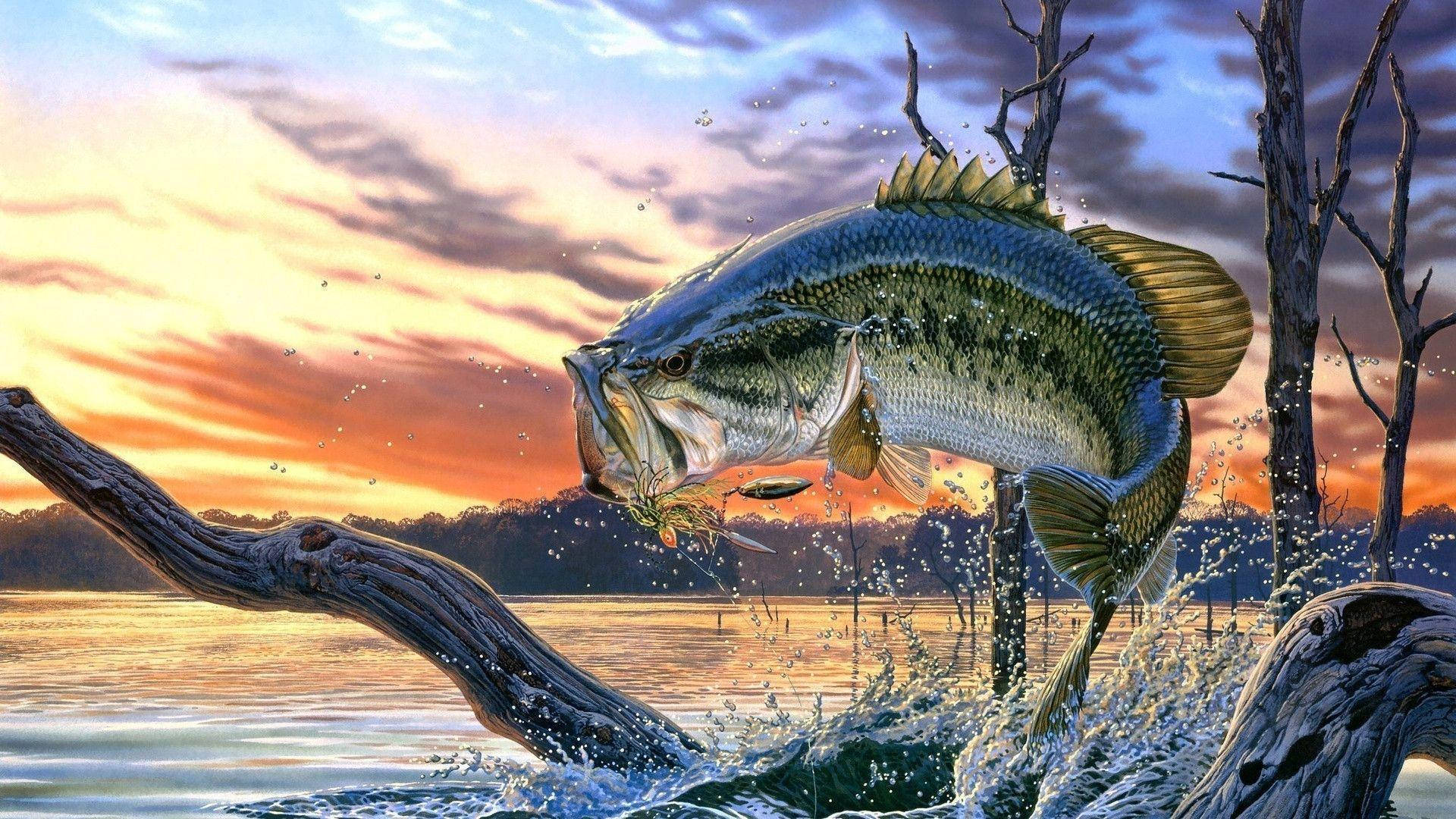The image depicts a highly detailed and possibly AI-generated scene of a largemouth bass dramatically leaping out of the water, seemingly in the midst of a fight, gripped by a spinnerbait lure in its open mouth. The fish, characterized by its green and white coloration and intricate markings, is captured in dynamic motion, with its tail curled towards its head and water splashing vividly around it. In the foreground, an old, twisted piece of driftwood extends from the bottom left corner to the middle of the scene, adding to the rustic aesthetic.

The backdrop features a serene lake mirroring a stunning, multicolored sunset, blending hues of smoky orange, purple, light blue, and yellow, and is framed by distant mountains and possibly sparse trees. The sky is a harmonious composition of dark clouds and vivid sunset tones, all reflected in the calm surface of the lake, enhancing the image's tranquil yet vibrant atmosphere. The combination of detailed elements and lifelike textures highlights both the serene beauty of nature and the raw power of the jumping bass, making the image captivating and full of vitality.